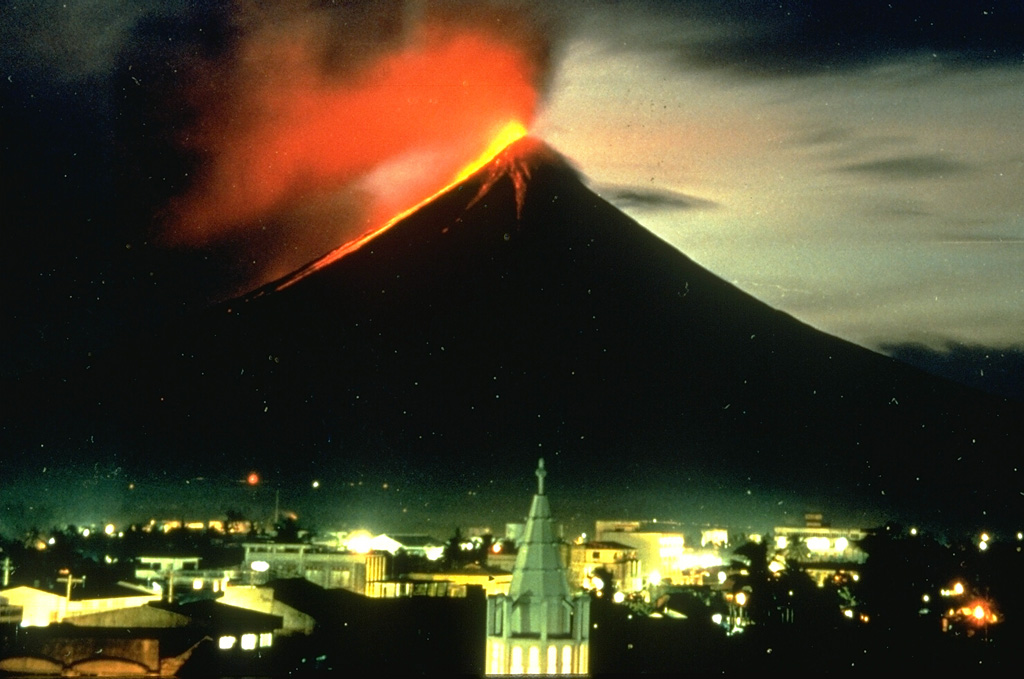This captivating and vintage photograph captures a dramatic nighttime volcanic eruption. The towering, black, triangular volcano dominates the background, with vibrant orange lava and flame-like yellow streams cascading down its slopes. The sky is an evocative mix of smoky gray and glowing orange-red hues, possibly illuminated by the eruption itself, suggesting the event occurs just after sunset or before sunrise. The left side of the sky shows dense black clouds mixed with orange clouds, while the right side has a brighter, bluish tinge with a dark black cloud in the upper right.

Below the menacing volcano lies a quaint city, likely Japanese, characterized by its small buildings and traditional architecture. The city's focal point is a prominent church steeple, crowned with a triangular roof and a cross. The city's lights twinkle against the dark night, highlighting the contrast between the serene, illuminated foreground and the chaotic, fiery spectacle of nature in the background.